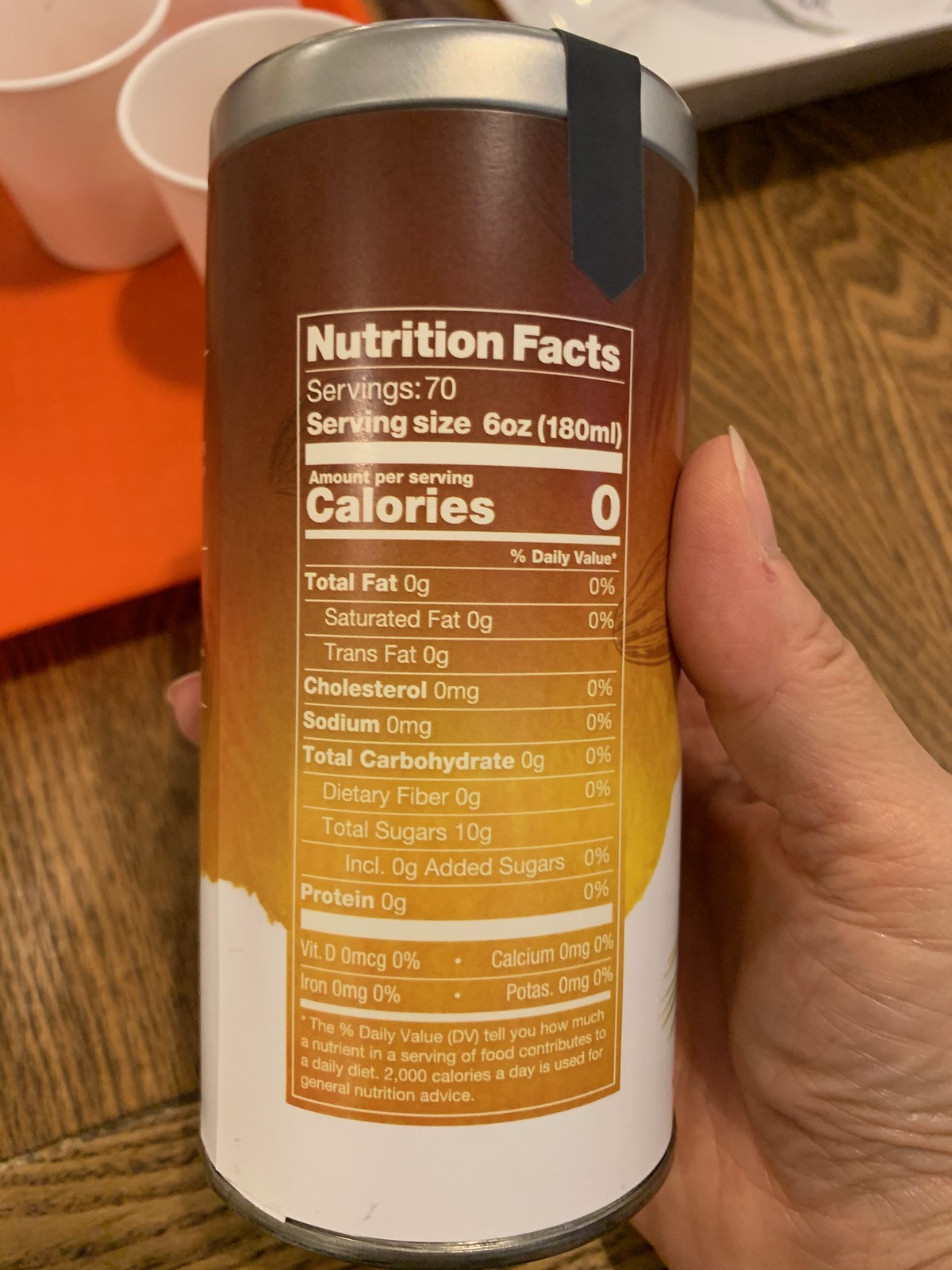The image features a person's right hand, palm side up, holding a canister that shifts in color from brown at the top through light brown to white at the bottom. The canister has a silver top with a black tab, and prominently displays nutritional facts on the back. These details include 70 servings, each with a serving size of 6 ounces (180 milliliters), zero calories, zero fat, zero cholesterol, zero added sugars, and various vitamins and minerals listed. Surrounding the canister is a wooden table with a couple of paper cups on an orange placemat, and a metal object off to the right, suggesting it might be used for preparing a beverage, possibly a powdered drink mix.